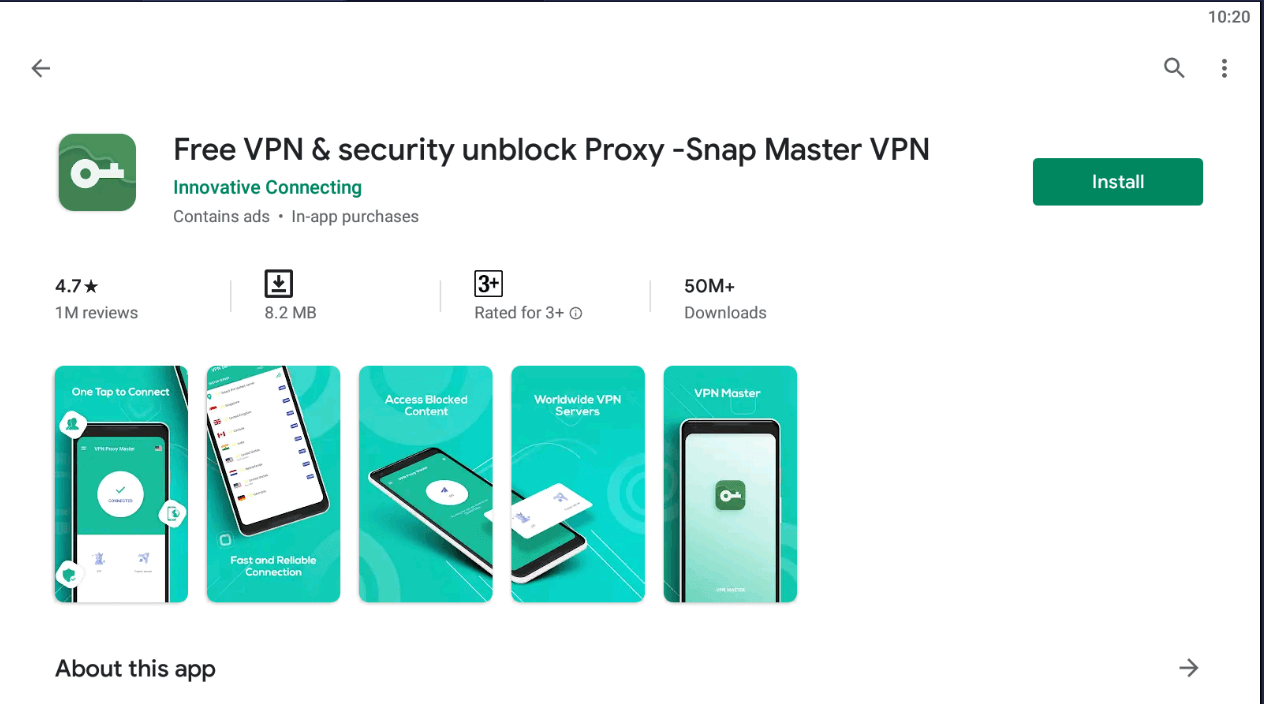The screenshot displays the app page for "Free VPN and Security Unblock ProxySnap Master VPN" on a digital platform with a white background. Central to the image is the app's title displayed in prominent green text, accompanied by a small, square logo with rounded corners featuring a white key on a green background. Below the title, the text "Innovative Connecting" is written in green, with a note in small gray text indicating "Contains Ads · In-App Purchases."

To the right of the title, there is a green rectangular button with the word "Install" in white, suggesting that clicking it will install the app on the user's device. Above this button, there are several key app statistics. The first is a 4.7-star rating with a black star symbol, and nearby, it notes "1 million reviews." Other icons show a download icon followed by "8.2 MB," indicating the app's size, and a square icon labeled "3+," denoting the recommended age suitability. The far right shows a download count of "50M+," reflecting over 50 million downloads.

Dominating the lower portion of the screen are five greenish-blue simulated windows showcasing various features of the app. At the very bottom of the screenshot, the phrase "About this app" is written in black text.